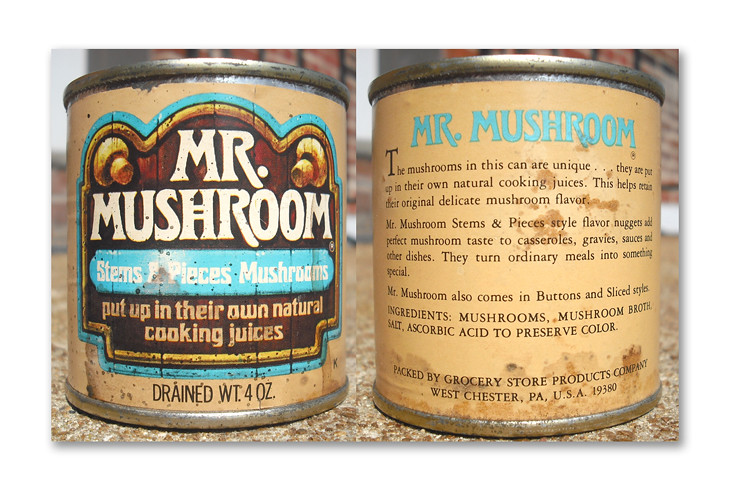In this image, the background features a blend of light gray and brown tones, with hints of a gray wall interspersed with brown elements. Dominating the foreground is a countertop with a mingled pattern of brown and white. Centrally placed on the countertop is a small aluminum can labeled "Mr. Mushroom," prominently displayed in white text on a brown background with a light blue outline. A blue banner on the can announces "Stems and Pieces Mushrooms" in white text. Below this, there is additional text in light brown that reads "Put up in their own natural cooking juices." The can also indicates a drained weight of 4 ounces. The back of the can, visible in the image, contains detailed information about the mushrooms.